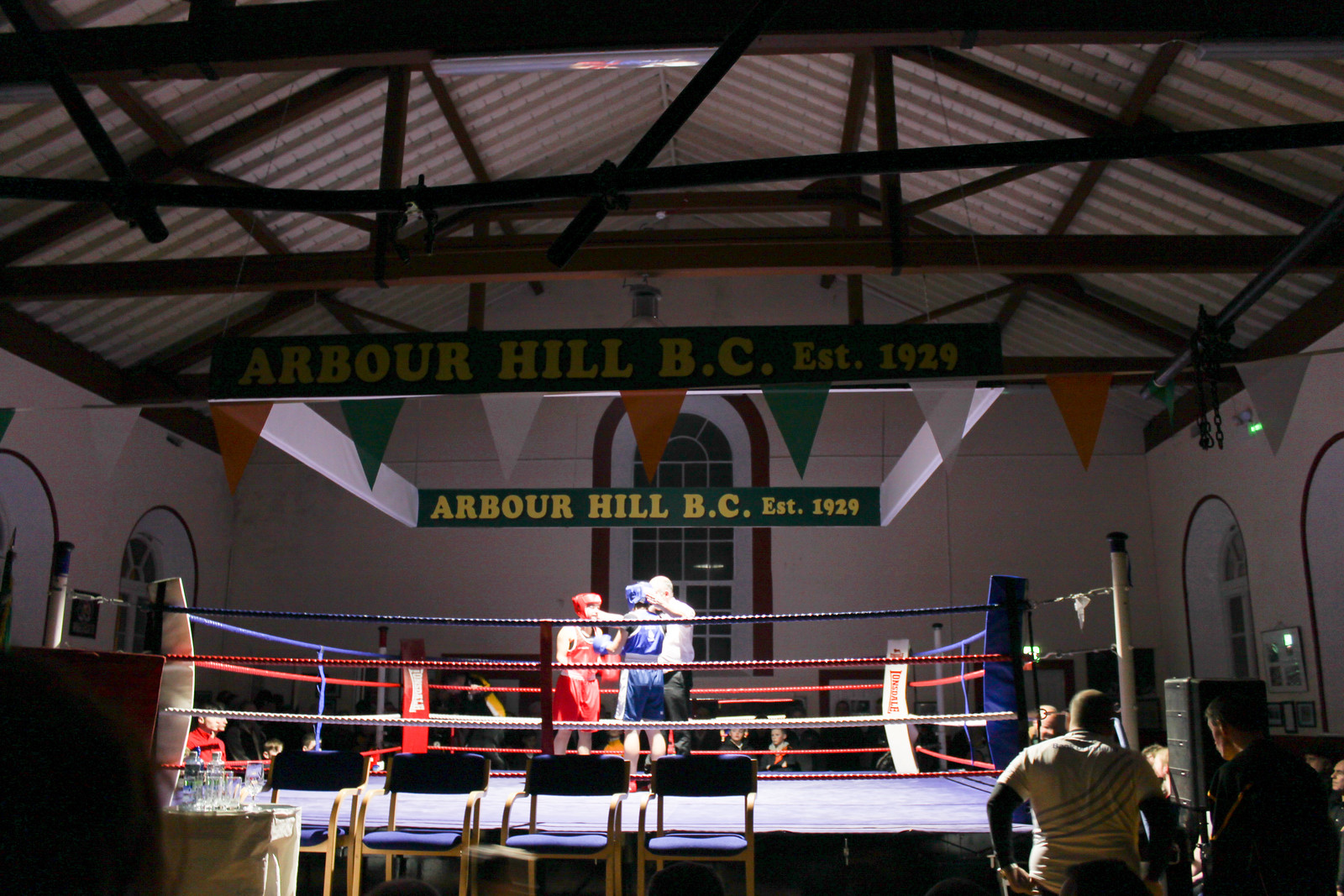In this image, captured from a distance, the scene centers on a boxing ring adorned with four ropes in blue, red, white, and red again, situated in the middle of a room. The ring is the focal point, and within it, two boxers, one in red and the other in blue, face each other, ready to spar. An official, dressed in black pants and a white short-sleeved shirt, stands nearby. The background features a prominent sign reading "Arbor Hill BC EST 1929" in yellow or orange text against a green backdrop, positioned above the ring. Surrounding the ring are stacked chairs and a small group of onlookers, including three or four children and several adults, suggesting this might be a training session. The lighting casts a spotlight on the two boxers, enhancing the intensity of the moment.